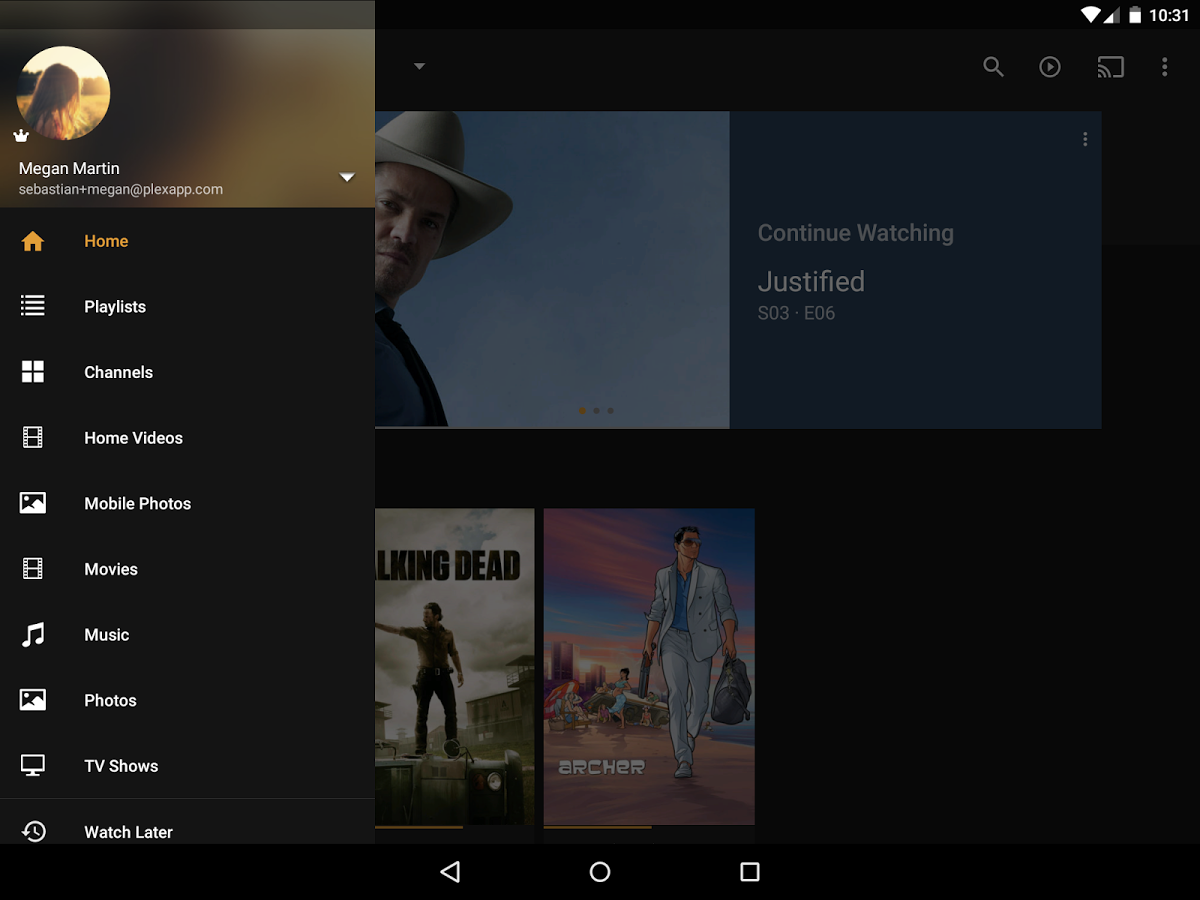A detailed cell phone screenshot displays the screen at 10:31 (either a.m. or p.m. is unspecified), showing a battery level indicator, cell tower signal, and Wi-Fi signal in the upper right corner. Below that, on the left side, a circular profile picture of a woman labeled "Megan Martin" is displayed, accompanied by a small crown icon symbolizing a premium or notable account. The text "Sebastian + Megan at FlexApp.com" appears under her name. 

Down the left sidebar, the options listed include Home, Playlists, Channel, Home Videos, Mobile Photos, Movies, Music, Photos, TV Shows, and Watch Later. On the right side of the screen, the "Continue Watching" section is visible, highlighting "Justified Season 3, Episode 6," with an image of a man in a cowboy hat. Below, previews of "The Walking Dead" and "Archer" are also visible.